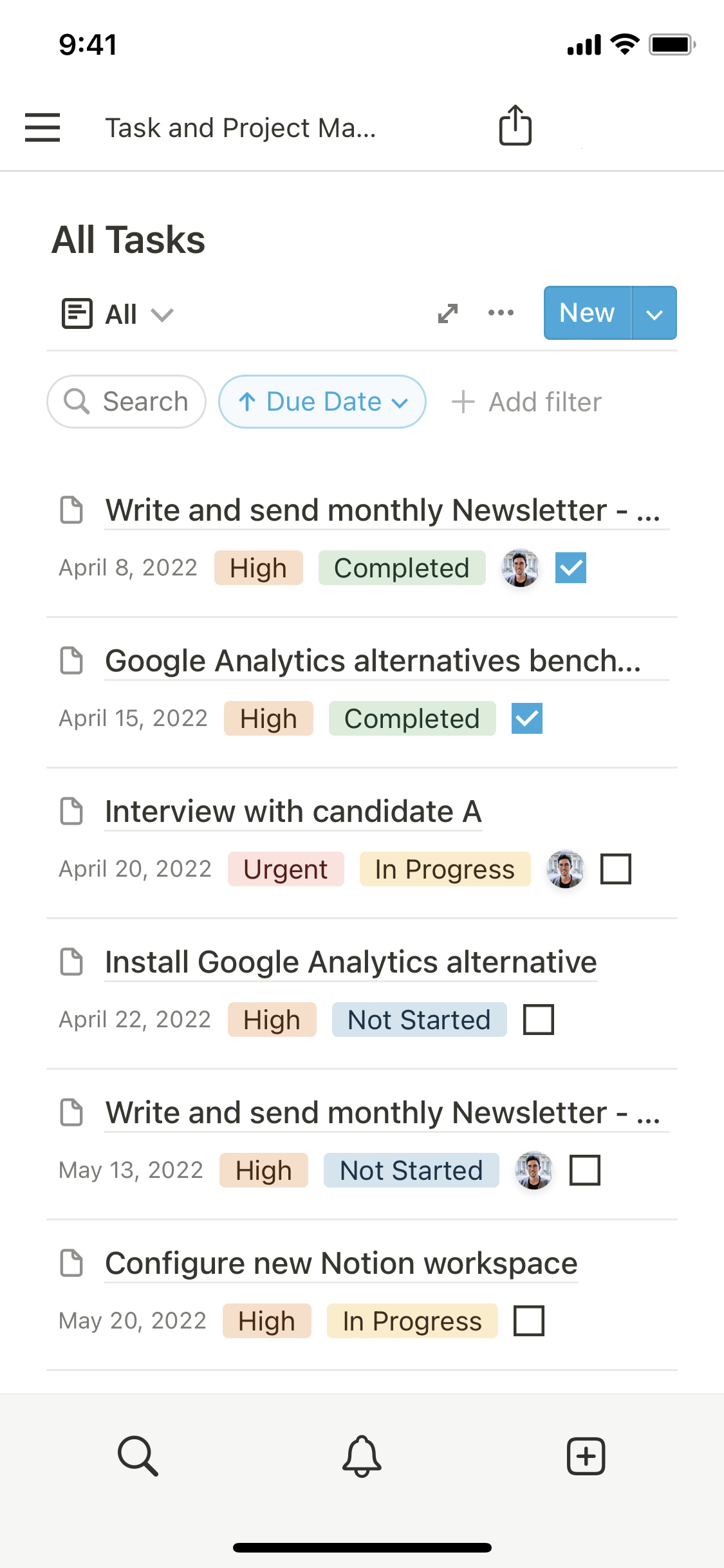The image is a screenshot of a cell phone displaying a task management application against a pure white background, which seamlessly blends into the surrounding area. The image is approximately three times as tall as it is wide. 

At the top left corner of the screen, the time is displayed as 9:41 AM. On the upper right, there are full signal strength icons and a fully charged battery indicator. 

Just below, on the left side, there is a menu icon consisting of three horizontal bars. To the right of the menu icon, small black text reads "Task and Project Ma...", likely short for "Management". A solid gray line follows, delineating the header from the content below.

The main content area begins with a bold, black header on the left that says "All Tasks". Directly beneath this header, there is a dropdown menu labeled "All" with a downward-facing arrow, indicating filter options. Adjacent to it, there is a search bar and a toggle button for organizing tasks by due date. Further to the right, there is a plus sign labeled "Add Filter," allowing users to add additional filters to their task list.

The task list itself shows six tasks:
1. "Write and send monthly newsletter"
2. "Google Analytics alternatives bench..."
3. "Interview with candidate A"
4. "Install Google Analytics software"

Each task is listed one after the other, providing a clear, organized view of pending activities.